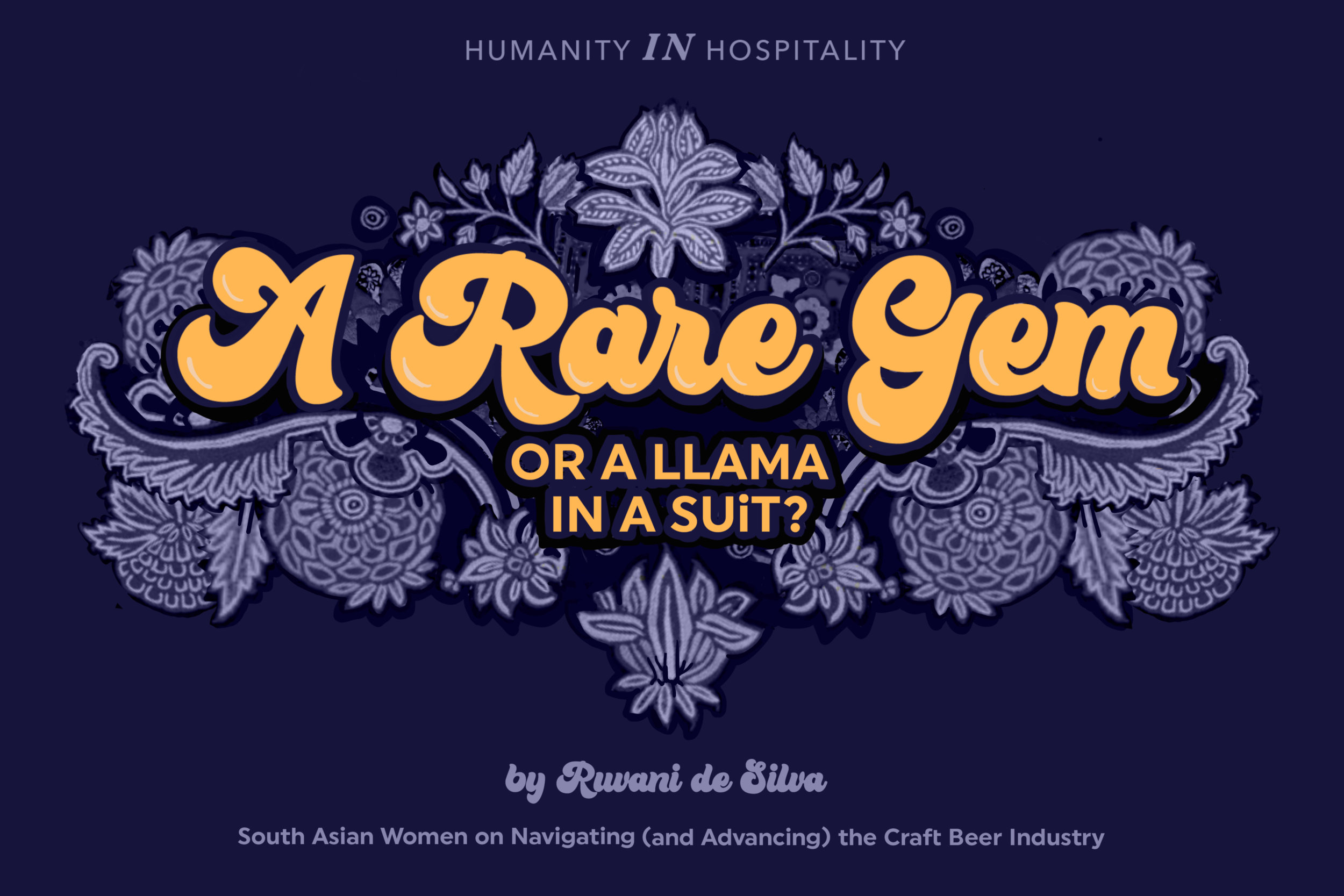The poster features a dark, indigo-blue background with intricate, light-purple floral designs embellishing the layout. At the very top center, in bold, light-purple letters, it reads "Humanity and Hospitality." Below this, a more detailed floral pattern frames the central section where, in vibrant yellow-orange letters, it says "A Rare Gem" followed by another phrase, "or a llama in a suit." Towards the lower portion of the poster, the name "Juani De Silva" is elegantly written in script. Finally, at the bottom in smaller light-purple font, it states, "South American women are navigating and advancing the craft beer industry," with "and advancing" enclosed in parentheses.